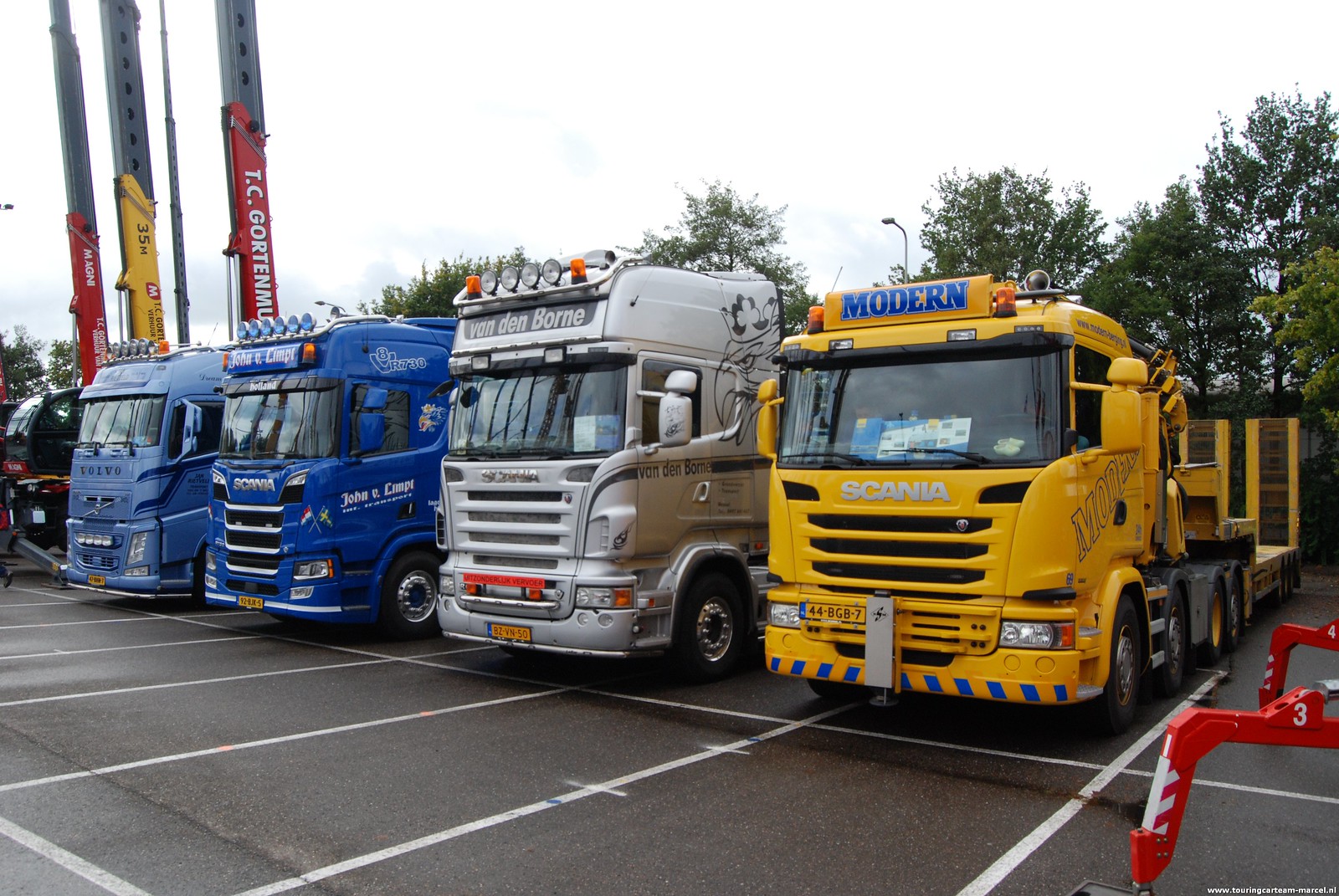This photograph depicts a parking lot exhibiting an array of utility trucks parked side-by-side, viewed from an eye-level angle. Starting from the left, there is a yellow truck adorned with a blue modern Texas emblem and the text "35M” and a red symbol. Adjacent to it is a silver truck bearing the inscription "Texas Van de Born" in white. Further along, two blue trucks with white text are visible, behind which additional trucks are partially obscured. Notably, several trucks feature large crane-like arms extended vertically into the sky; one bears the name "T.C. Gorton," and another arm displays the term "M-A-G-N-I." Various makes, including Volvo and Scania in blue, silver, and yellow, are evident, with one blue truck displaying a brochure on its dashboard. This setup, possibly indicating a truck show, appears on a drizzly day, as discerned from the slightly muted lighting and wet surface, lending a peculiar charm to the scene.